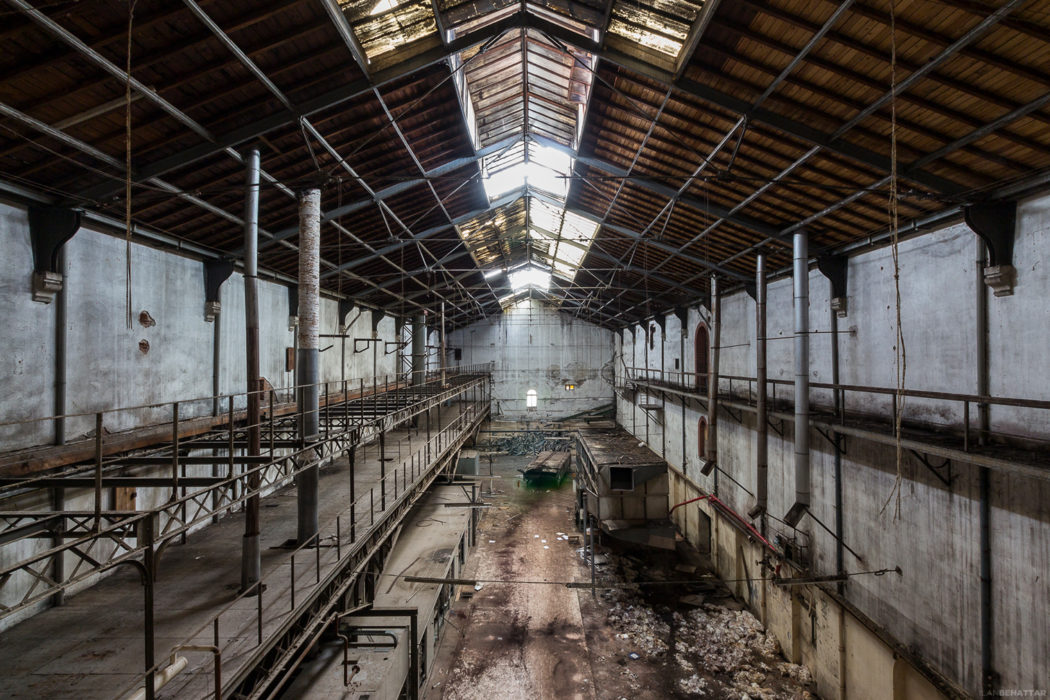This color photograph captures the interior of an old, abandoned factory building, taken from an elevated perspective at one end. The once-industrial space is now empty and shows signs of significant degradation, with debris scattered across the dirty, brown floor. A mixture of steel and iron pipes hang from the raised ceiling, some extending down the sides and others crisscrossing the space, adding to the visual chaos. The ceiling itself has gaps where some roof panels are missing, allowing natural light to filter in, and features windows in the middle that partially illuminate the desolate scene. On the left side, a second-level walkway is visible, lined with more pipes, while to the right, another walkway can be seen, accompanied by what appear to be old cabinets. The walls, likely made of concrete, further emphasize the building’s industrial past, now overshadowed by its worn-down, fire-damaged appearance.